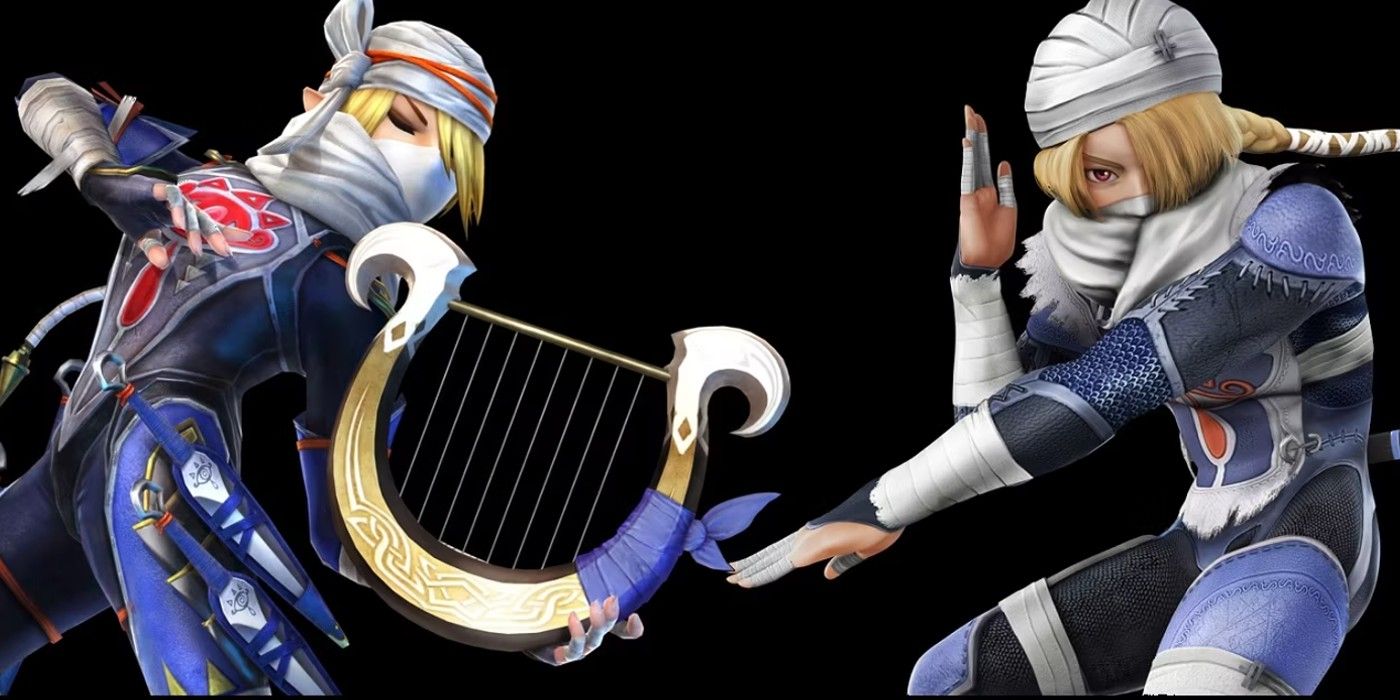This detailed, computerized image features two stylized warrior characters, reminiscent of video game graphics, possibly depicting elves. Both characters have blonde hair, pointed ears, and are dressed in modern ninja-like outfits with a mix of blue, black, and gray colors, accented by white, yellow, and red details.

The left character sports a blue and gray outfit with red accents, including a notable red logo on the chest, white bandages around the right forearm, and an orange-striped headband. This character holds a gold and white harp in a poised yet relaxed manner.

The right character, akin to the first in attire and appearance, strikes a dynamic martial arts pose with their left arm directed towards the image's bottom middle and their right arm raised with a flat hand. Both characters have masked faces and wear white shawls or scarves around their necks, adding a mysterious, coordinated element to their ensemble. The image is set against a black background, and no text is present, enhancing the striking visual focus on the characters.